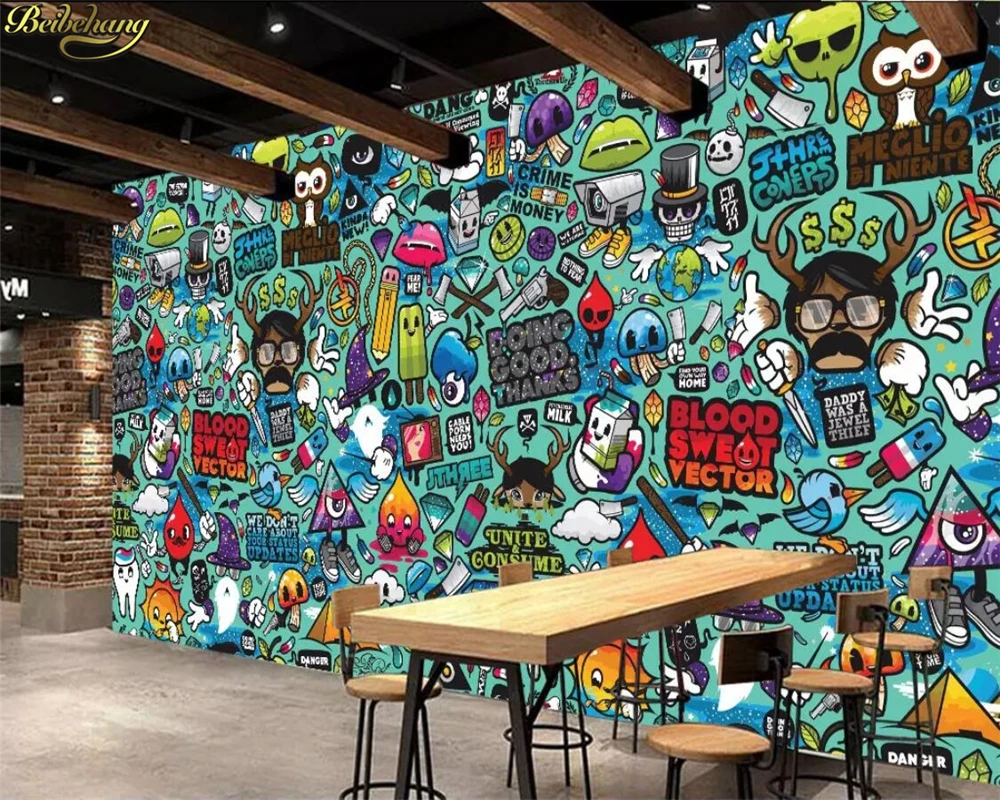This photograph captures a vibrant wall mural inside a bar or restaurant. The mural, set against a seafoam green background, features a repeating design of a cartoon man with glasses and antlers, surrounded by animated hands holding various objects like a knife and cash, and throwing gems. Alongside this central figure, the mural includes an eclectic mix of doodles such as an owl, a milk carton, lips, a man with horns, a mushroom with a knife, a drop of blood, a gun, a diamond, two intersecting X's, a pencil with a happy face, a popsicle with a happy face and hands, and a triangle with an eye. Phrases like "blood, sweat, vector" and "doing good things" are interspersed throughout the mural. In front of this colorful tableau stands a wooden table surrounded by four round stools, with a concrete gray floor beneath and a brick column to the left. The ceiling features dark brown beams extending into the wall, enhancing the room's eclectic and artistic ambiance.